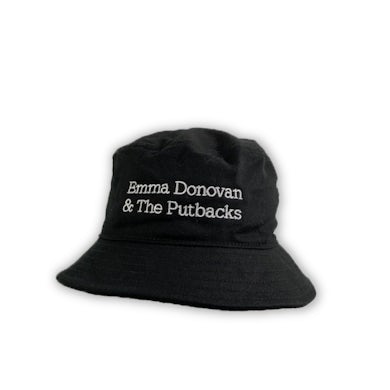This photograph features a black bucket-style hat with a soft, slightly crinkled fabric, indicating it has been worn multiple times. The hat has a continuous brim encircling it, which appears somewhat stiff, likely designed to keep the sun out of the wearer's eyes. Displayed prominently on an all-white background, the hat shows a small shadow underneath, adding a subtle depth to the scene. The most distinctive feature of the hat is the white text stitched on the front above the brim, which reads, "Emma Donovan and the Putbacks," contrasting sharply against the black fabric. This simple yet detailed image showcases the hat centered perfectly with a clean and focused presentation.